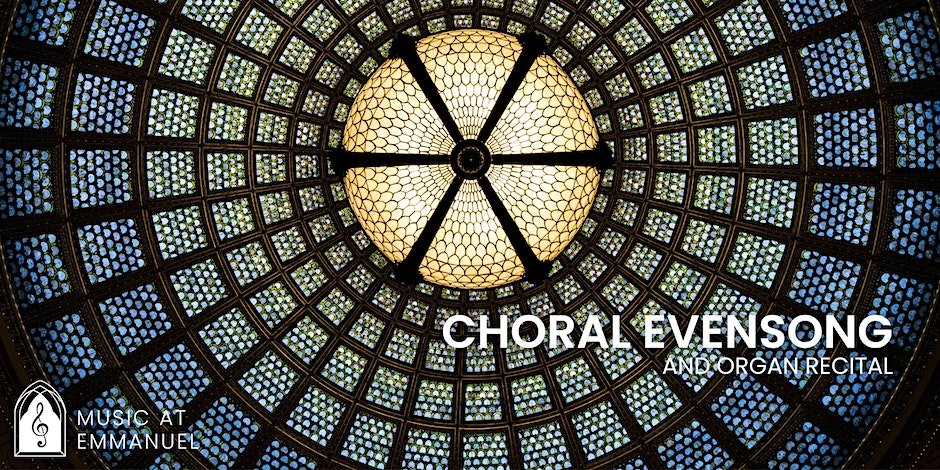The image showcases the intricately designed ceiling of what appears to be a church or an orchestra hall. Dominating the scene is a grand, sun-like chandelier or light fixture, encased in an elaborate metal framework. Lines radiate outward from this central fixture, creating a symmetrical, circular pattern adorned with numerous small blue windows, each framed in black webbing, forming a grid-like design. The overall aesthetic suggests careful architectural planning, possibly to enhance the acoustics of the space. The bottom corners of the image contain text, with the bottom left featuring a headstone-shaped icon, inscribed with the words "Music at Emmanuel" and a music note, while the bottom right announces an upcoming event: "Choral Even Song and Organ Recital." The blending of these elements creates a visually striking and complex scene, hinting at an elegant venue prepared for a sophisticated musical performance.